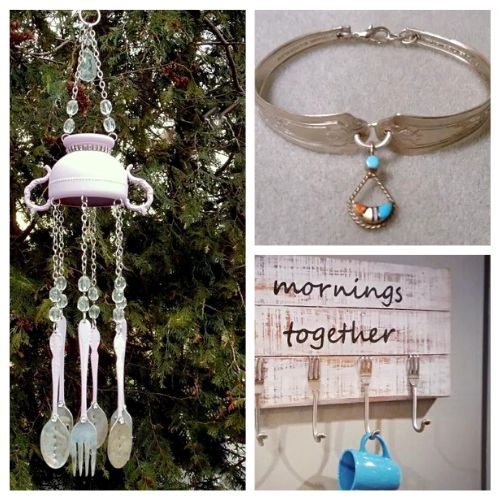This is a detailed Instagram post featuring a three-part visual arrangement of photographs showcasing various decorative household items. The leftmost image is a vertically-oriented photograph depicting an ornate outdoor wind chime set against a backdrop of lush green trees. The chime includes an upside-down teacup with handles and a string of hanging utensils—forks and spoons with pink handles—that add a whimsical touch to the outdoor setting.

In the upper right corner, there is a close-up of a beautifully crafted bracelet. The bracelet appears to be made of silver with a turquoise stone and other semi-precious stones incorporated into its pendant, giving it a distinctive, possibly Native American, aesthetic.

The bottom right image portrays a wall-mounted wooden cup holder made from weathered, whitewashed wood. The board is inscribed with the phrase "mornings together" in black script. The cup holder itself features hooks fashioned from the handles of forks, three of which are empty, while the second hook from the right holds a charming robin's egg blue mug.

Together, these images meld the detailed intricacies of handmade jewelry and home decor into a cohesive and visually engaging collage.